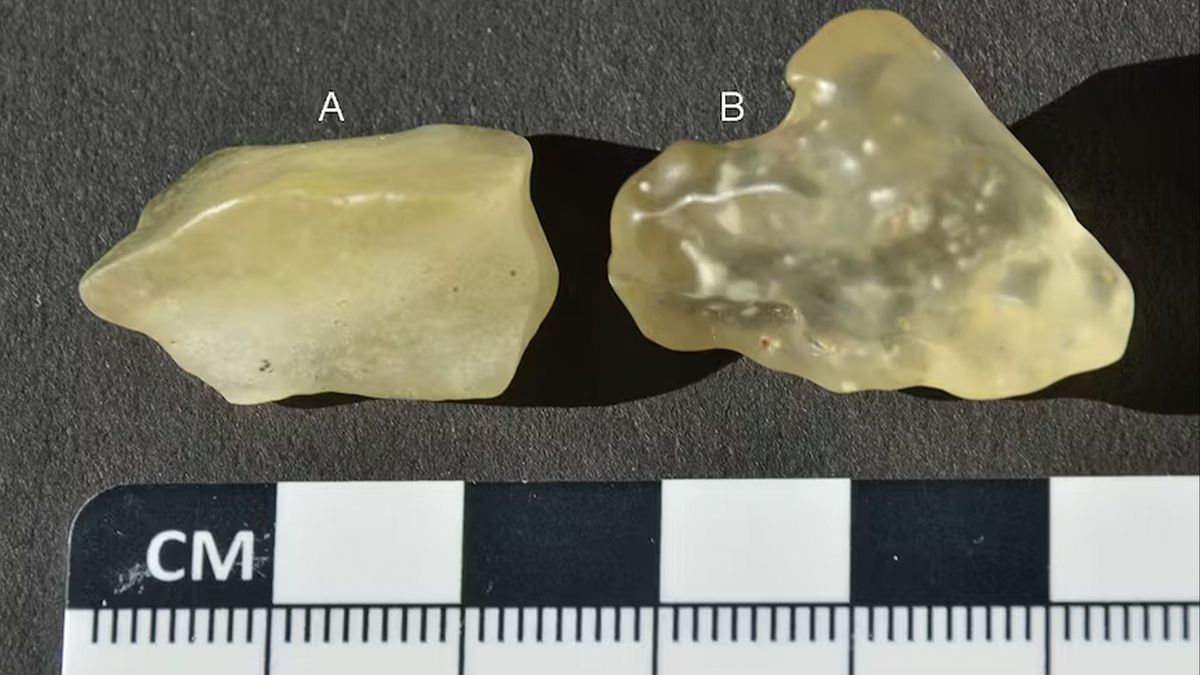This photograph displays two irregularly shaped, translucent gemstones or crystals positioned on a dark gray background. The stones, which exhibit a pale yellow hue with a whitish tinge, are labeled with white letters: 'A' for the stone on the left and 'B' for the one on the right. Stone 'A' appears as an off-white color and smoother in texture, while stone 'B' is slightly more jagged and more translucent. Both stones cast shadows to their right. Below the stones, a black and white checkered ruler marked in centimeters (indicated by the letters 'CM' in white) provides a scale, suggesting that each stone is approximately 2 to 3 centimeters in width. The gemstones seem to be in their natural, unpolished form, possibly hinting at a setting related to jewelry or archaeology.